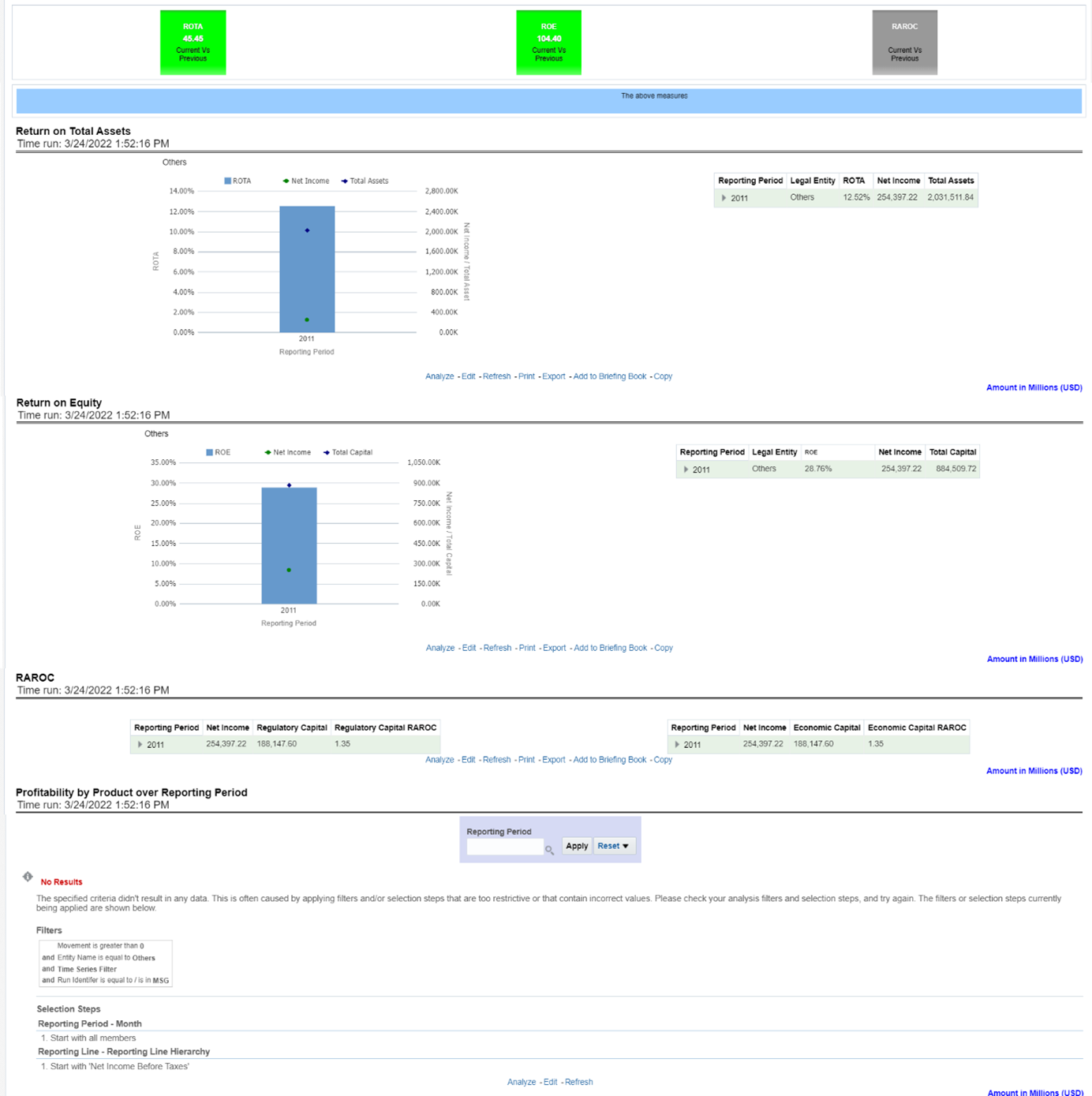**Detailed Caption:**

The image displays a detailed financial dashboard. The upper portion of the screen is predominantly white, featuring three distinct boxes on the left side. 

- The first box, located on the far left, is green with white text that reads "ROTA 45.5." Below this, in black text, it states "Current vs Previous."
- The second box, centrally positioned, is a vibrant green. It contains white text indicating "ROE $104.40," followed by "Current vs Previous" in black.
- The third box on the right is gray with white text displaying "RAROC" and "Current vs Previous," but it lacks a numerical value.

Directly beneath these boxes is a blue strip centered with the text "The above measures." 

The lower portion of the screen is mainly white. It includes the text "Return on Total Assets" along with a timestamp reading "3-24-2022 1:52 p.m."

Below this text, a chart is presented, featuring a blue bar graph. The graph is labeled "ROTA" on one side, with percentages on the vertical axis starting at 0% and increasing by increments of 2% up to 14%.

The entire setup provides a comprehensive visualization of financial performance metrics.